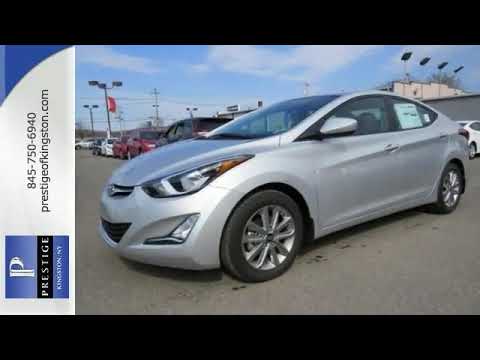This is an outdoor photograph of a silver 4-door sedan in a parking lot, possibly taken for an advertisement. The car features a rounded top, front headlights, silver wheel covers, and a decal in the back window detailing information about the car or its pricing. The scene includes several other cars behind it, suggesting the location might be a car dealership lot. The concrete parking lot is grey, and a commercial building with lights is visible in the background. On the left side of the image, there's a vertical strip featuring the Prestige logo, including a blue, white, and black "P" icon, the location "Kingston, New York," a phone number (845-750-6940), and the website PrestigeofKingston.com.